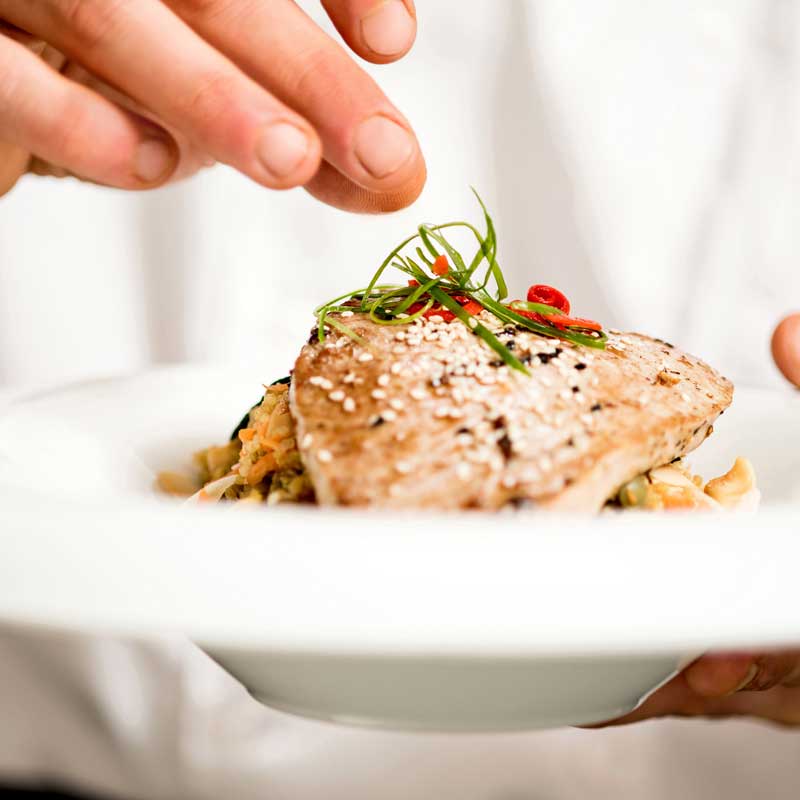This photograph captures a detailed, close-up view of a delectable chicken dish artfully presented in a white bowl. The bowl, which has a shallow depth akin to a deep plate, cradles a bed of vegetables, likely including carrots and possibly broccoli, with hints of white rice peeking through. Atop this base, a piece of carefully roasted chicken or possibly a thin, seared fish filet takes center stage, adorned with a sprinkle of white and black sesame seeds. Complementing the dish, delicate microgreens and a touch of red bell pepper or chili add vibrant color and sophistication.

Foregrounding the culinary craftsmanship, a white man's fingers are visible in the top left quadrant, meticulously placing the finishing touches of garnish. His other hand supports the plate from the bottom right side, steadying the dish. The background features solid white fabric, part of his chef’s outfit, suggesting a professional kitchen setting. The composition of the image, taken from an angle slightly below the hand level, adds a dynamic, intimate perspective to the chef’s presentation.